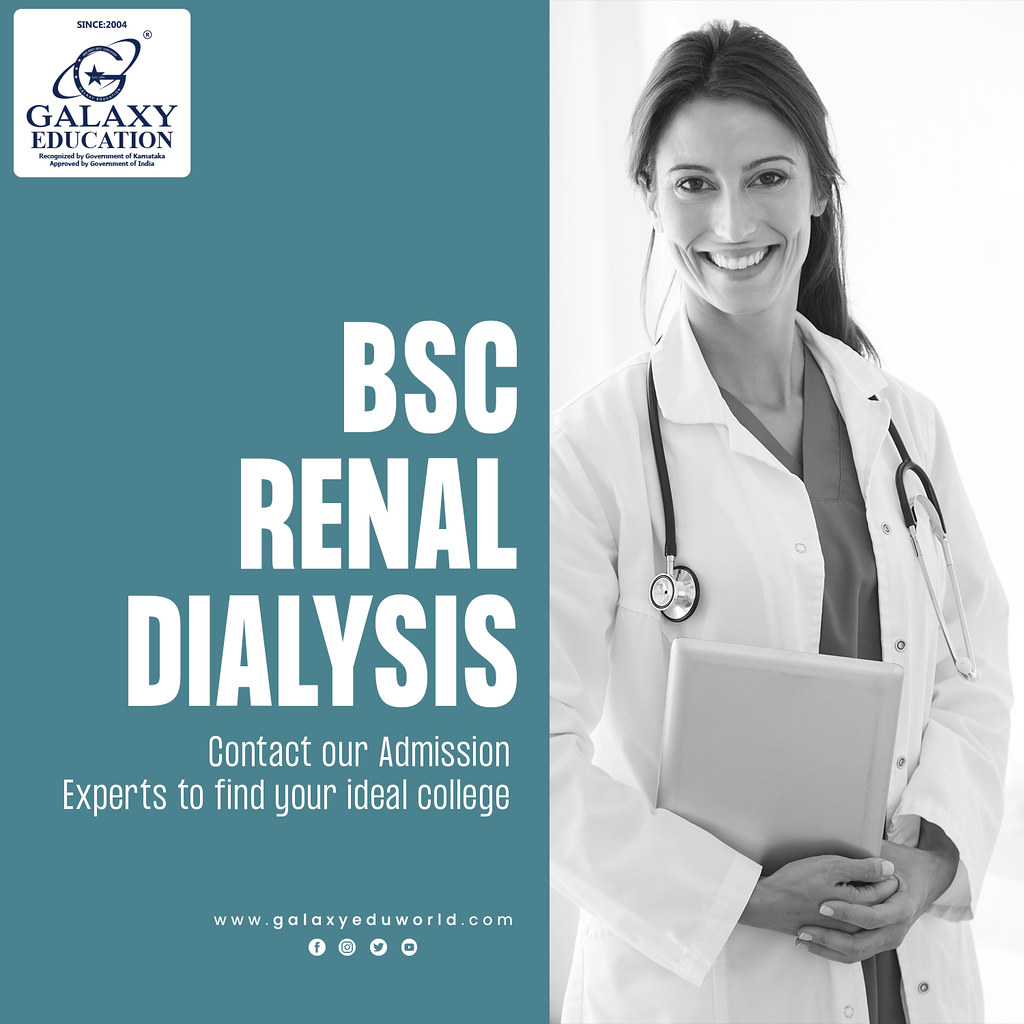An advertisement postcard features a striking design split into two sections: the left half is turquoise with bold white text, while the right half displays a grayscale image of a smiling female doctor. The doctor, with brown hair pulled back into a low ponytail, wears a white lab coat over scrubs and a stethoscope draped around her neck. She holds a booklet or folders in her hands. On the turquoise left side, large text reads "BSC Renal Dialysis" and "Contact our admission experts to find your ideal college." The upper left corner displays a white square containing "Galaxy Education since 2004" and a 'G' logo with a star. The bottom features the website www.galaxyeduworld.com and icons for Facebook, Instagram, Twitter (X), and YouTube within white circles.